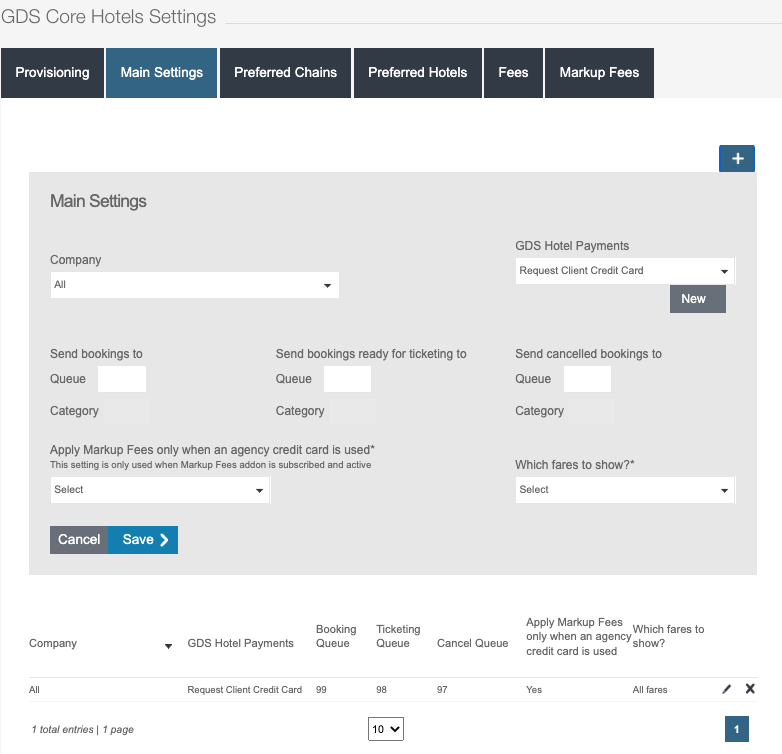The image displays a professionally designed yet simple website interface for "GDS Core Hotels Settings." The main header "GDS Core Hotels Settings" is positioned at the top left, with a gray horizontal line extending from the "S" across to the right side of the page. Below this, the site navigation menu includes options such as "Provisioning," "Main Settings," "Preferred Chains," "Preferred Hotel Fees," and "Markup Fees." Each menu item is enclosed in a black box, except for the "Main Settings," which is highlighted in a blue box, indicating it is the current selection.

The content area below the menu is predominantly white, featuring a prominent blue plus sign above a gray block labeled "Main Settings." This section contains various input fields and dropdown options for configuring settings. 

- "Company" is highlighted and has an associated dropdown arrow.
- "GDS Hotel Payments" includes a button labeled "New" for adding new configurations.
- Various fields specify where to send different types of bookings, such as "send bookings to," "send bookings ready for ticketing to," and "send canceled bookings to," each with corresponding dropdown selections.
 
Additionally, there are two positioned select boxes side by side with dropdown arrows for making selections. At the bottom of this section are "Cancel" and "Save" buttons, with the "Save" button featuring a right-pointing arrow. Finally, company information is displayed at the bottom of the page.

The structured interface ensures ease of navigation and accessibility for configuring hotel settings effectively.